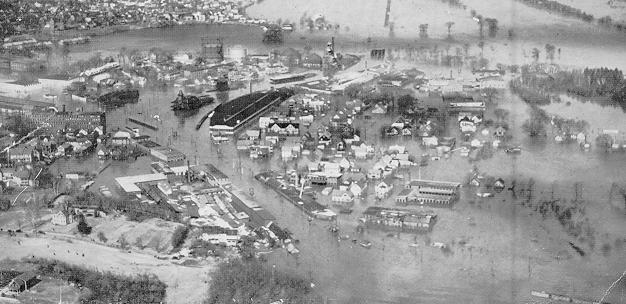This is a very old aerial black and white photograph capturing a city that appears to be severely flooded, likely due to a hurricane or an intense storm. The grayscale image depicts numerous buildings submerged halfway up in floodwaters, with water pouring in from the top right corner of the frame, suggesting the origin of the flooding. The photo, notable for its high vantage point and historical nature, shows a clear demarcation where the floodwaters cease, revealing dry land in the left-hand bottom corner, likely a higher elevation area. The cityscape is quite detailed, with visible trees scattered among the buildings, adding to the chaotic scene of a city overwhelmed by water.